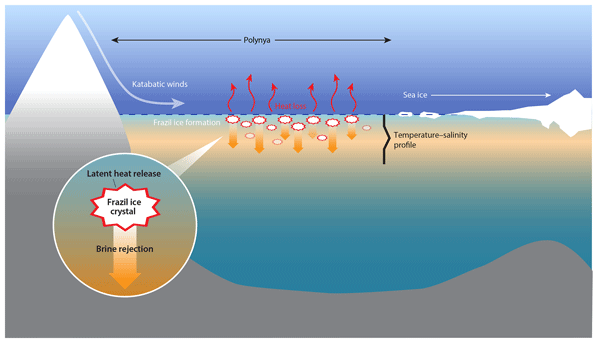This detailed, blue-toned educational illustration depicts the process of sea ice formation and the interactions of winds and temperature changes. In the center of the rectangular diagram, the term "Polynya" is prominently displayed, with arrows extending left and right, indicating the area where this phenomenon occurs. To the left, a peak represents a mountainous formation, from which arrows labeled "katabatic winds" flow downwards and towards the right. The diagram shows the interaction of these winds with the landscape and water.

Central to the illustration is a "Temperature Salinity Profile," marked by a black line dividing various zones of the water. Above the water's surface, red arrows indicate "heat loss" while pointing upwards, denoting the escape of latent heat into the atmosphere. The water area includes further labeling of "frazzle ice formation," showing early ice crystals near the surface. Arrows labeled "brine rejection" point downwards from these crystals, depicting how salt is expelled during the formation of ice.

To the right side of the diagram, "sea ice" is indicated with a white arrow pointing to a mass of icy forms, providing a contrast to the adjacent mountainous area. The colors in the illustration are soft and gradient, creating a visually easy-to-read and simple layout. Underneath the water surface, further details like white circles with red borders denote specific processes, all contributing to the comprehensive explanation of the interactions between wind, temperature, and ice formation.